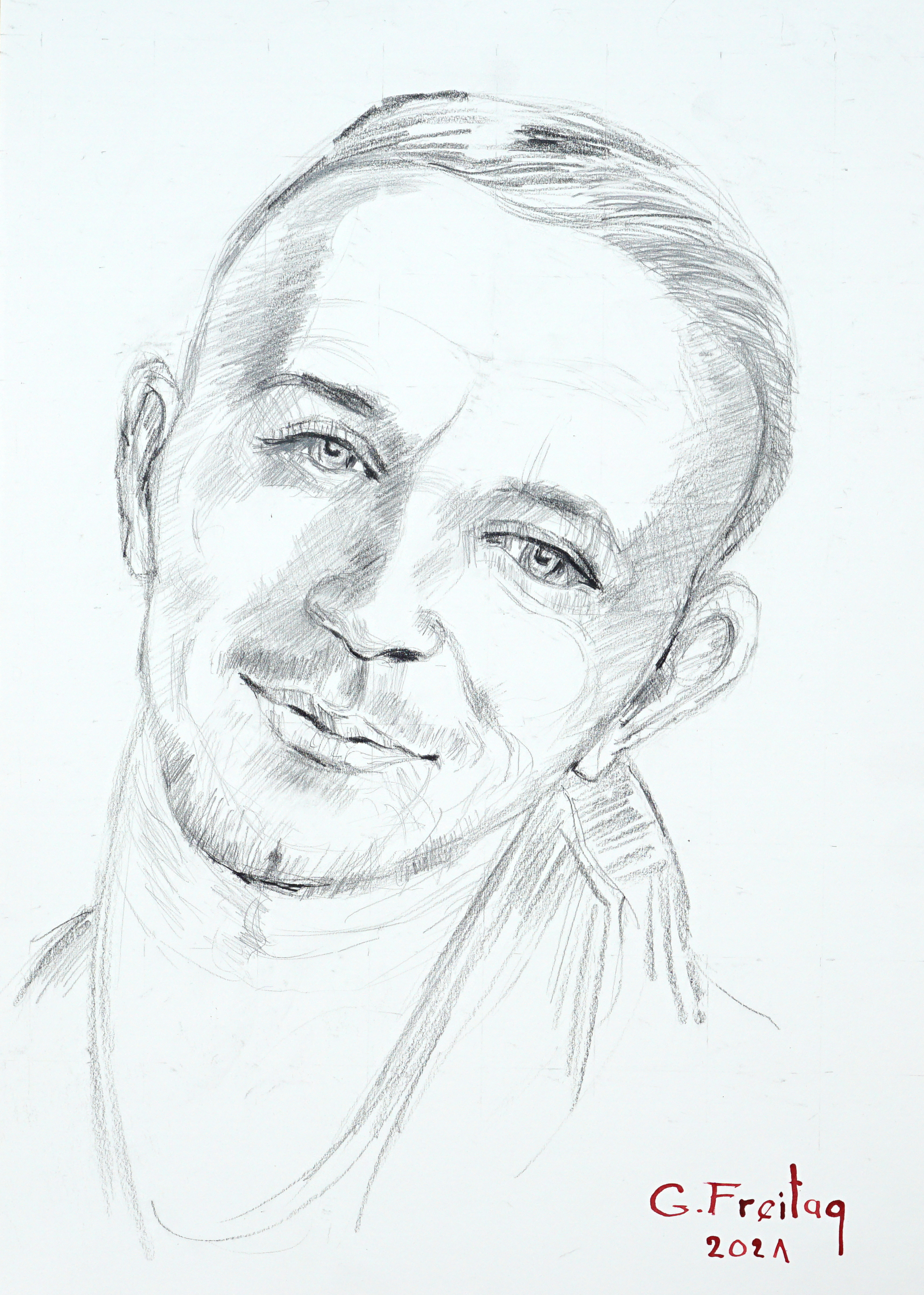This detailed pencil sketch, signed "G. Freytag, 2021" in red ink at the bottom, depicts a man seemingly in his 40s. The drawing is distinguished by a range of shading techniques, particularly crosshatching around the eyes and down the left side of the nose, giving it depth and texture. The man's short hair, possibly indicative of a receding hairline, is lightly shaded, suggesting a medium color. His eyes, drawn with darker lines, exude a contemplative, perhaps slightly sad expression, as he glances downward. The man's facial features include some light wrinkles around the eyes and forehead, a dimpled chin, sparse mustache, and a bit of beard growth. He wears a T-shirt and his head is subtly tilted to the right, with his neck slightly bent, adding to the overall impression of introspection. The sketch is set against a light grey background, emphasizing the detailed pencil work that captures the nuanced emotions of the subject.